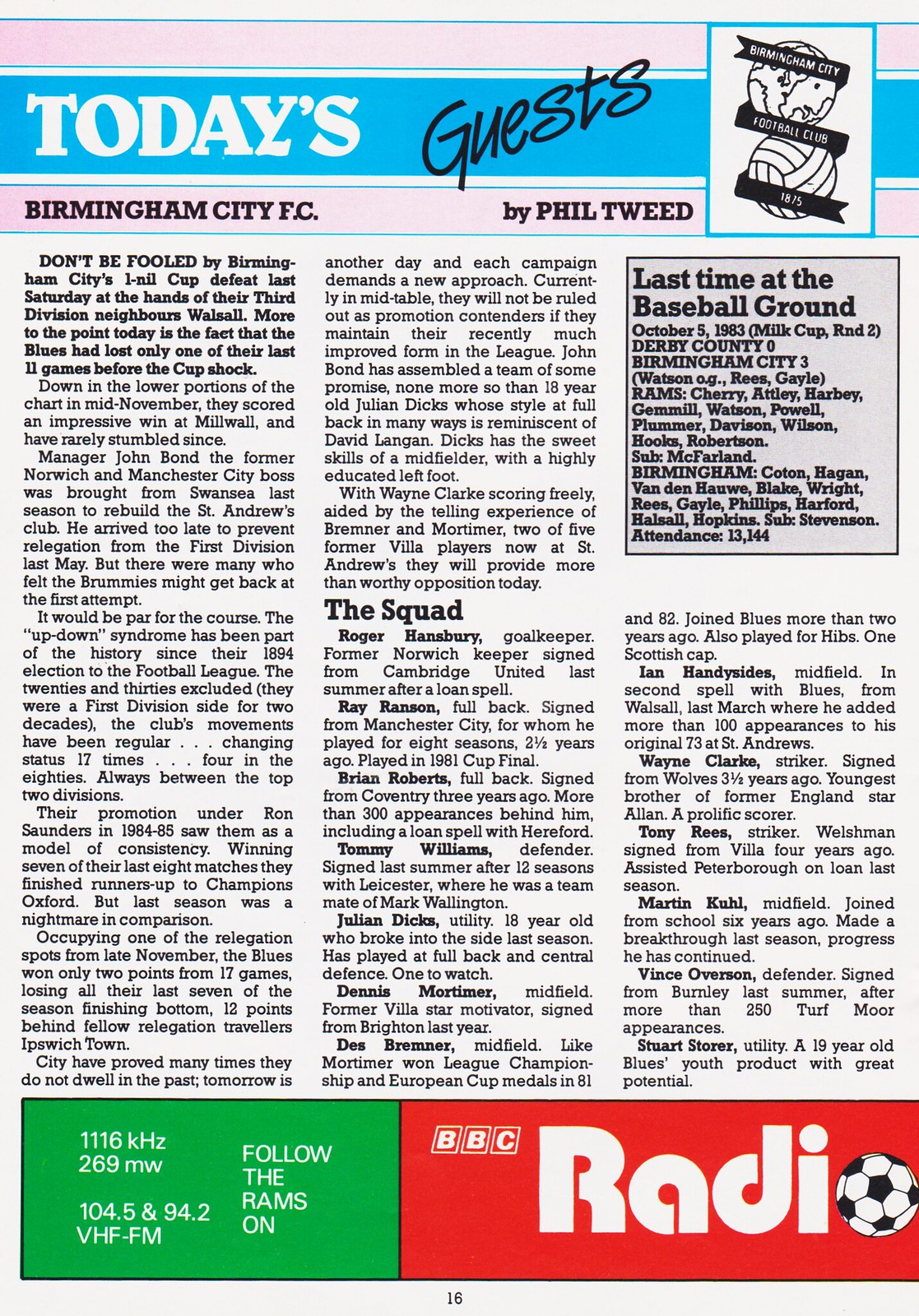This image features a detailed page from a game day program or sports publication centered around Birmingham City FC. The header of the page showcases a distinct design with pink, blue, black, and white elements, and includes the title "Today's Guests" alongside the Birmingham City Football Club logo. This logo displays two soccer balls with a ribbon running through them, inscribed with "Birmingham City Football Club 1875." The article beneath the header is by Phil Tweed and is divided into three columns of black text against a white background. 

The text begins with, "Don't be fooled by Birmingham City's 1-0 cup defeat last Saturday at the hands of their third division neighbors, Walsall. More to the point today is the fact that the Blues had lost only one of their last 11 games before the cup shock." The second column transitions to a subheading titled "The Squad," profiling approximately 14 players. In the top right corner of the third column, a small gray box contains historical text about a previous match: "Last time at the Baseball Ground, October 5, 1983, Milk Cup Round 2, Derby County 0 Birmingham City 3."

The footer of the page, featuring green and red elements, promotes BBC Radio with frequency information: "1116 kHz, 269 MW, 104.5, and 94.2 VHF FM," and a red banner reading "BBC RDI" alongside a black and white soccer ball graphic.